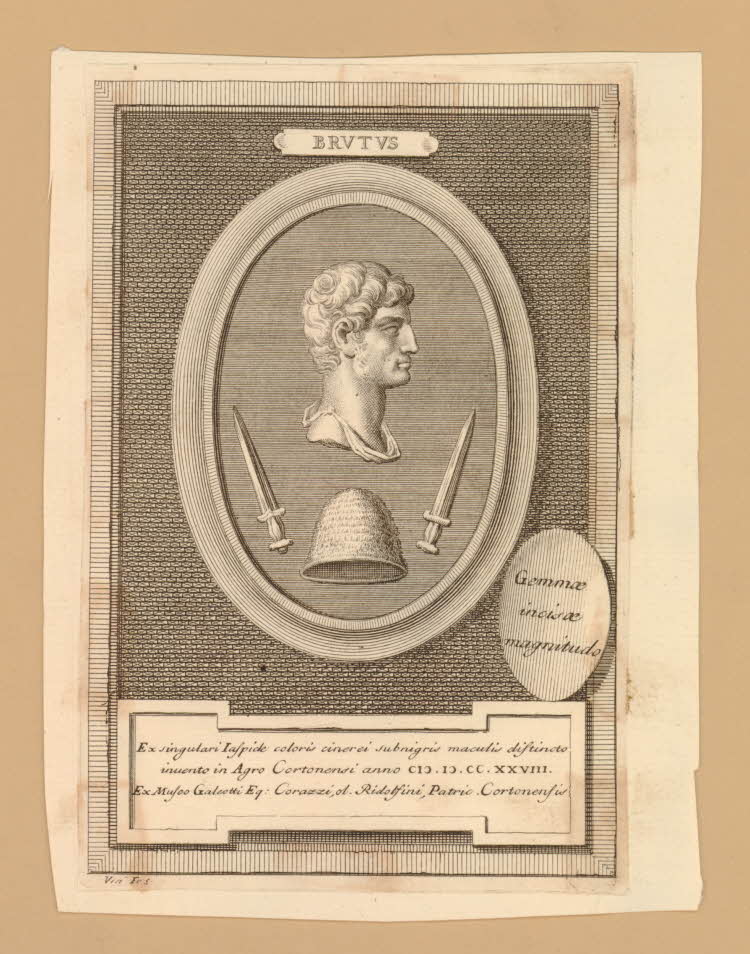The image is an aged depiction of a historical page, resembling an ancient Roman stamp or drawing, with a darkened white, off-white appearance that accentuates its old-fashioned, line-art style. At the top of the image, within an oval frame, the title "BRVTVS" is displayed, featuring Roman-style typography where the 'U's appear as 'V's. Central to the image is a man's head, presumably Brutus, looking towards the right. Directly below his head is an antiquated helmet, distinctly resembling an upside-down bowl. Flanking the helmet are two small, vintage Greek-style daggers. To the side, another oval contains the Latin phrase "Gemae incisei magnitudo," with additional unreadable Latin text below. The entire scene is set against a tan, textured background, enhancing the image's historical feel.